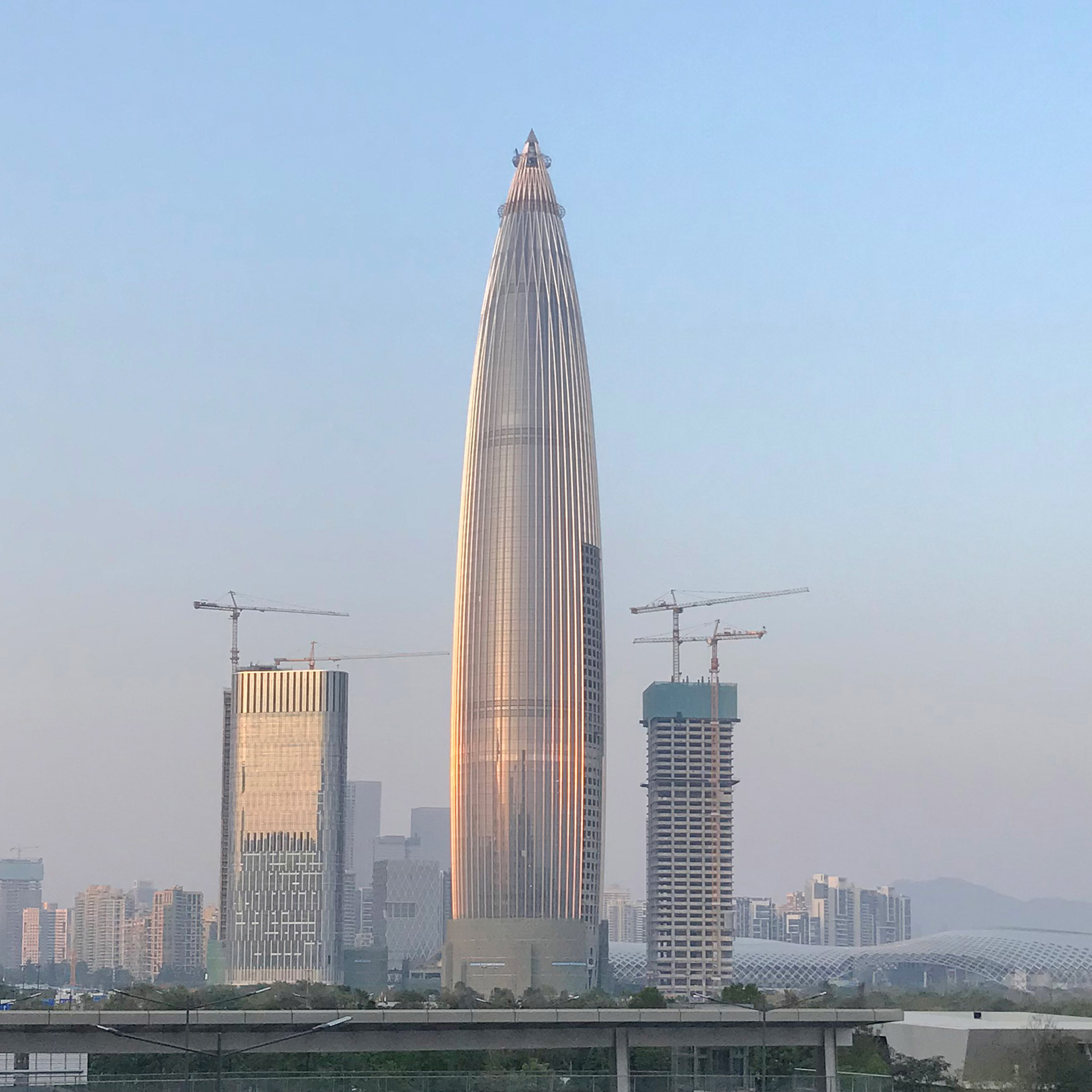This photograph captures a striking cityscape shrouded in haze, possibly taken during dawn or dusk. Dominating the center of the frame, a towering, cylindrical skyscraper with a tapered top and reflective glass windows stands prominently, flanked by two slightly shorter skyscrapers on either side. Each of these flanking buildings is crowned with two cranes, indicating ongoing construction. The upper two-thirds of the image showcases a hazy, light blue-gray sky, enhancing the mystique of the scene. In the foreground, a smaller building and possibly a bridge are visible, with sets of streetlights and sparse trees dotting the background. The overall impression suggests a vast, modern cityscape, potentially in Dubai, filled with additional buildings receding into the misty distance.